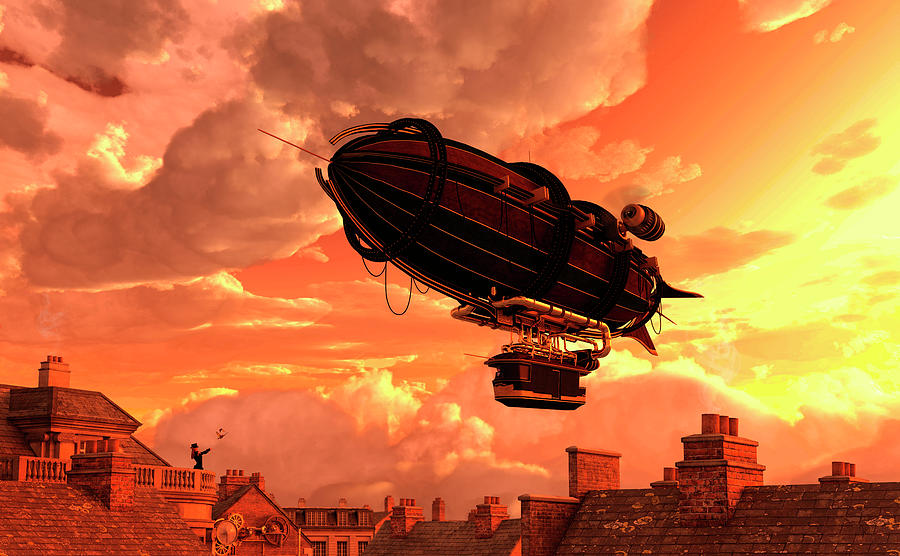This detailed illustration captures a fanciful scene dominated by a sleek, black blimp floating in the sky. The artwork is vividly rendered with a dreamy palette of yellow, pink, and orange hues, creating a stunning sunset backdrop with beautifully textured clouds. The scene looks almost surreal, possibly AI-generated, with its high realism. Beneath the blimp, a sprawling array of city rooftops stretches out, some of which have balconies. On one such balcony, a woman appears to be tossing something towards the blimp. Another figure, possibly a man, stands at the front of the structure beneath the blimp. The whole scene evokes a sense of nostalgia, reminiscent of an early 20th-century setting, enhanced by the old-school architectural elements. This breathtaking image melds romanticism and whimsy, inviting viewers to lose themselves in its captivating details.